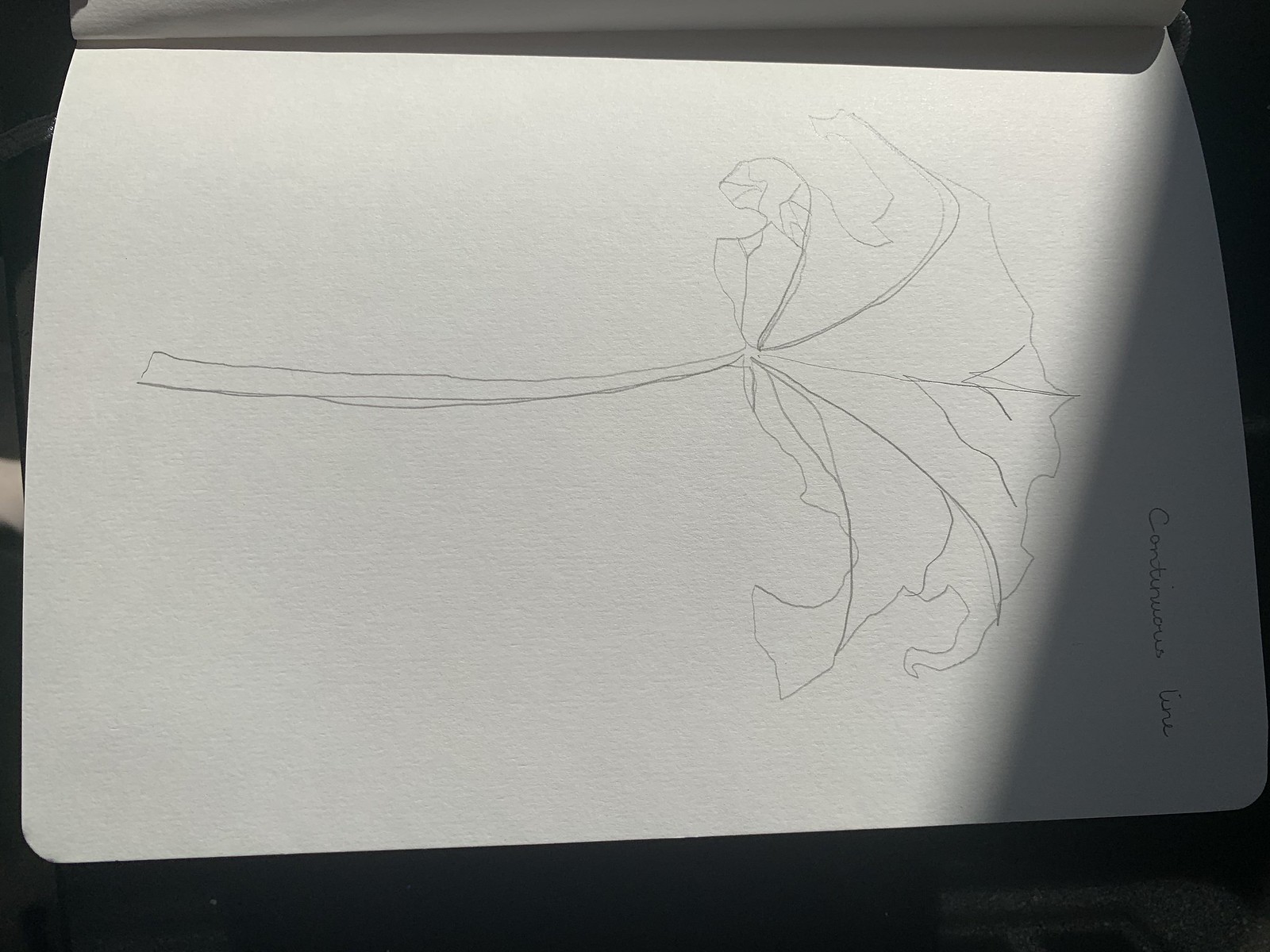In this photograph, we see a detailed pencil sketch of a leaf stem on a horizontally positioned sheet of paper. The sketchbook occupies nearly the entire image, which is framed with a dark background, contrasting sharply with the white page. The page itself, appearing in the upper portion of the image, curves slightly at its top edge, indicating it is from a booklet that is flipped open. The leaf depicted showcases intricate details, including the veins extending from the main stem and the pointed, ridged edges of the leaf itself. On the right side of the page, faint writing is visible in a shaded area, but the words "continuous line," written in cursive, stand out clearly, reinforcing that this sketch was drawn using a continuous line technique.